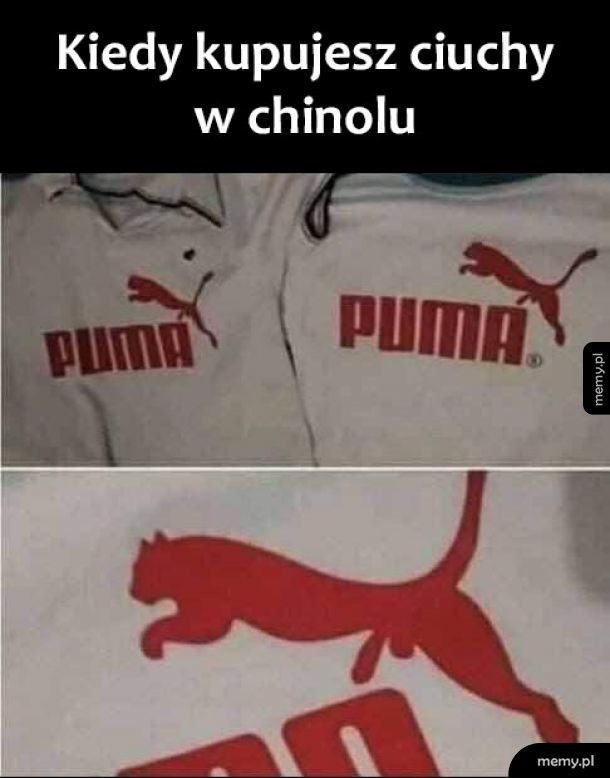The image is a rectangular collage divided into three main sections. The top section features a black background with white text in an unrecognized language, displaying the words "Kiri, Kupujesh, Shihuchi, W, Chinolo". Below the text, the middle section contains two images of a white garment, presumably a shirt or jersey. The first image shows the full garment with the Puma brand name and logo in red, featuring a jumping puma. The second image is a close-up of the Puma logo, which is notably different from the typical design, as it appears to show the puma's genitals. This alteration seems to be the focal point, likely intended as a humorous meme. Additionally, the website "memy.pl" is prominently displayed twice, once on the bottom right and again on the middle right, both against a black background.